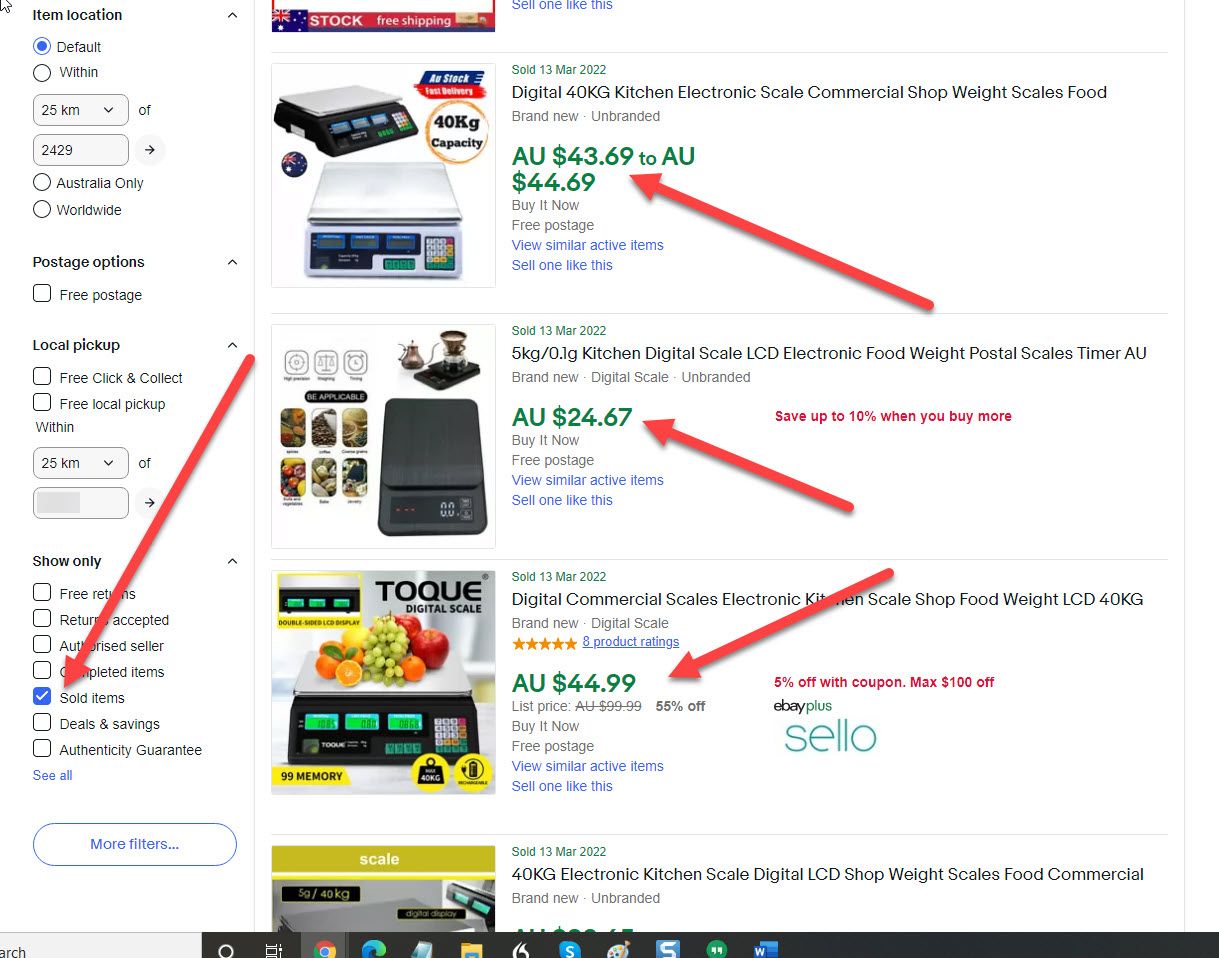The image appears to be a screenshot of an eBay search results page for various kitchen scales. Here is a detailed caption:

"The screenshot showcases eBay listings for kitchen scales, featuring diverse options suitable for culinary and commercial use. Prominently displayed are three complete listings, with hints of additional incomplete listings at the edges. At the top, there's a 'Digital 40 kg Kitchen Electronic Scale' suitable for commercial shop use, priced between AU $43.69 and AU $44.69, available with a 'Buy it Now' option and free postage. This item is noted as brand new and unbranded, and the sale date is visible. The image displays two scales: one in white and one in black.
Below this, a '5 kg/0.1 g Kitchen Digital Scale' with an LCD display intended for food and postal weighing is featured. The scale is available in black, and the listing mentions a discount of up to 10% for bulk purchases.
The next listing highlights a TOK digital scale, adorned with colorful fruit for illustrative purposes. Additional red arrows accentuate each product listing.
On the left side of the page, various filters for refining eBay search results are visible, including options to filter by item location, postage options, and local pickup. The 'Show Only Sold Items' filter is prominently checked in blue, accompanied by a red arrow pointing towards it."